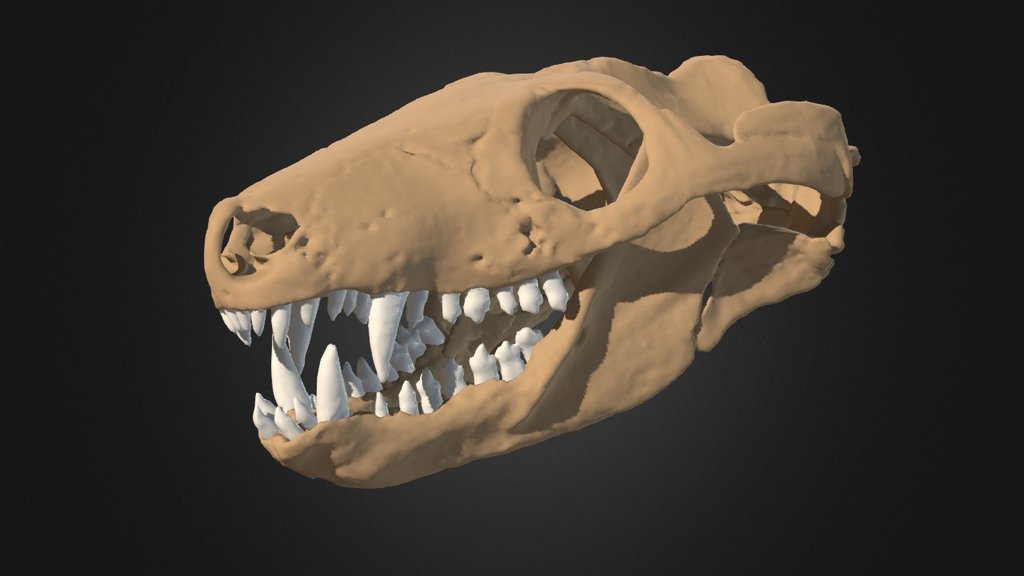The image depicts a computer-generated rendition of a dinosaur skull, quite likely that of a T-Rex, given its distinctive features. The skull is tan in color, with an elongated shape and sharp, dagger-like white teeth that are exceptionally well-preserved, indicating the CGI nature of the image. The eye sockets are boldly cut out, and the nasal openings contribute to its lifelike detail. A large ridge of bone adorns the back of the skull, suggesting space for significant muscle attachment, characteristic of predatory dinosaurs. The black background gives the impression that the skull is floating in space, further reinforcing the notion that this is a digital reconstruction rather than a physical model.